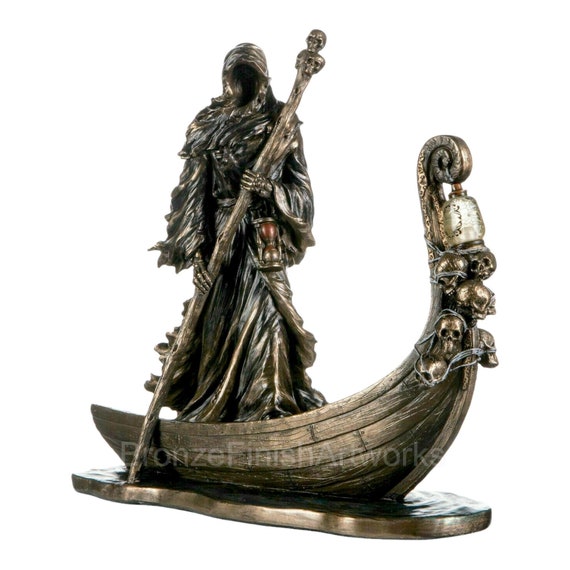This detailed bronze sculpture depicts the figure of Death, often referred to as Chiron, shrouded in a tattered, flowing cloak that obscures his face, creating a dark, eerie void beneath the hood. He stands in a weathered boat with a distinctive, Viking ship-like curved front, adorned with several skulls and topped with a lantern. This boat navigates what appears to be a bronze river. At his side, an hourglass hangs from his belt, tinged with a slight red hue, symbolizing the passage of time. Death holds a long staff, or what might be interpreted as an oar, ornamented with multiple skulls at the top, suggesting his journey across the mythical River Styx. His bony hands gripping the staff accentuate his skeletal, ghostly nature. The entire scene is highlighted with fine bronze detailing, adding to the sculpture's dark, majestic, and mystic aura.